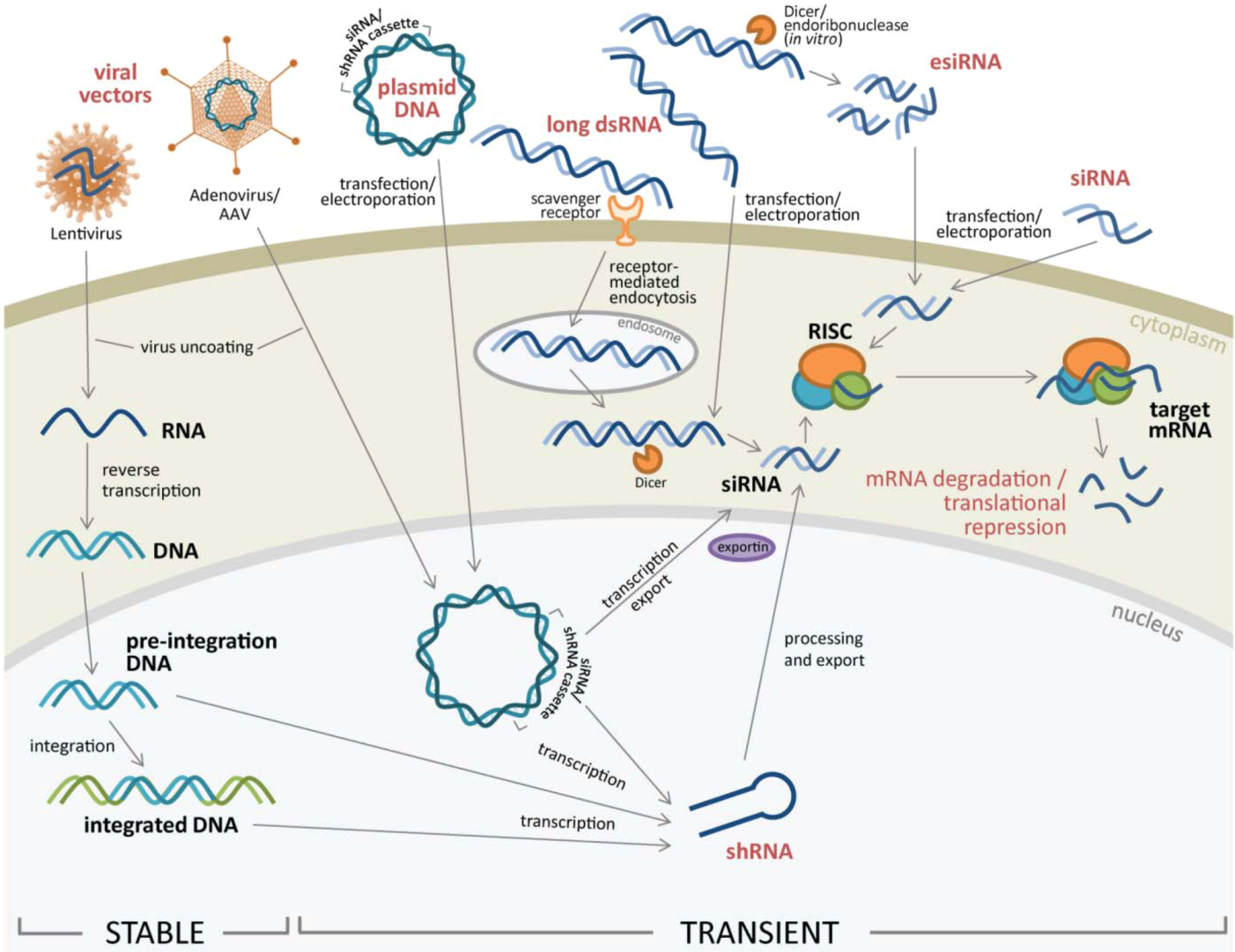This is a detailed scientific illustration of DNA and RNA relationships, spanning across three main horizontal layers and divided into sections labeled "stable" and "transient" at the bottom. The top part of the illustration features distinct lines representing different types of DNA and RNA, including plasmid DNA, long double-stranded RNA (DS RNA), and viral vectors. The viral vectors are visually depicted with a typical virus star-like icon, rendered in blue and orange colors.

In the central beige area, the diagram delves into processes involving RNA and DNA, highlighting transcription and the roles of various components like RISC (depicted in orange, blue, and green), which are associated with mRNA degradation, translation, and repression. Additionally, red SH RNA arrows point towards blue SI RNA, emphasizing their interconnected pathways.

The illustration also includes detailed representations of integrated DNA, pre-integrated DNA, and various forms of RNA, all interconnected by green and blue or purple squiggly lines. At the very bottom, further flows and movements of DNA are shown in a flowchart-like manner, distinguishing between stable and transient states to clarify their differences.

Notable terms scattered throughout the diagram include lentivirus, adenovirus, AAV, transfection, electroporation, target mRNA, nucleus processing, and export. This comprehensive and technical diagram effectively maps out the complex relationships and processes governing DNA and RNA in a visually structured format.